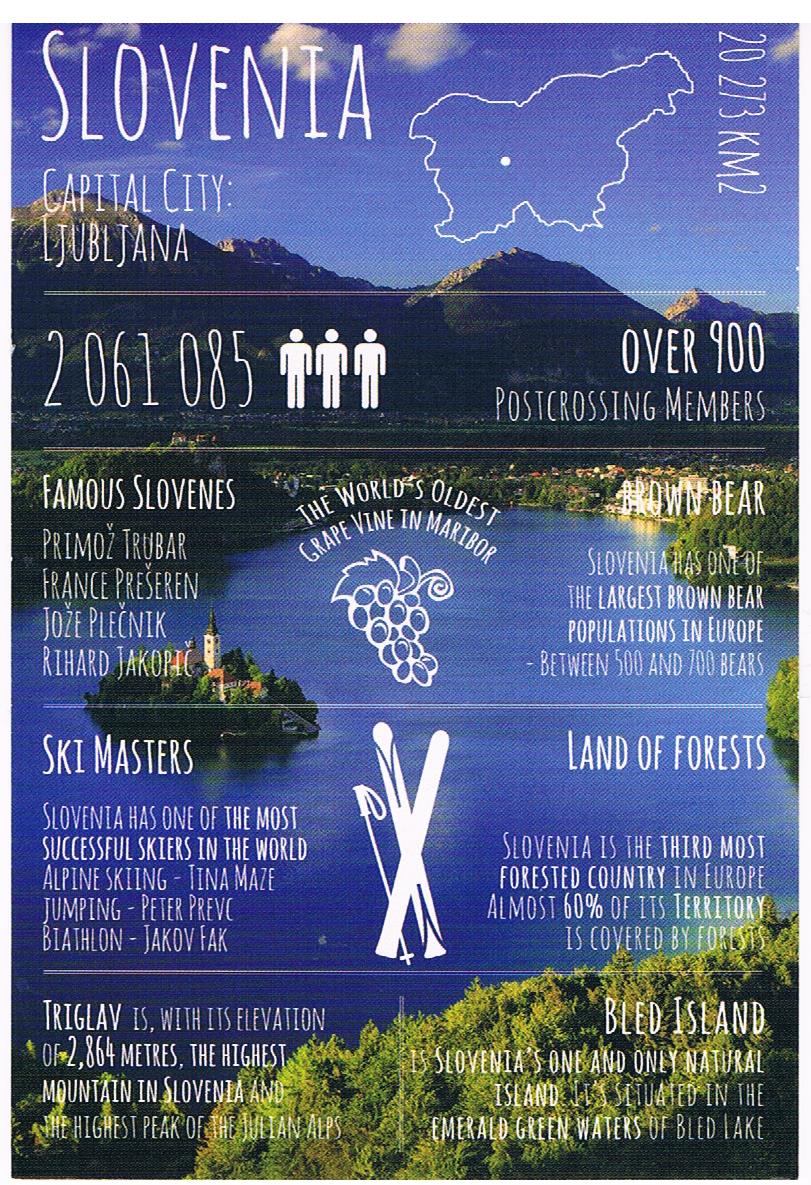The image is a detailed infographic promoting Slovenia, featuring an outdoor daytime scene dominated by a serene lake with an island castle at its center. Surrounding the lake, the landscape is rich with green forests and a town nestled in the background, framed by distant mountains and a blue sky filled with clouds. Overlaid on this picturesque scenery is white text providing various facts about Slovenia. 

In the top left corner, "Slovenia" is prominently displayed, followed by key statistics: the capital city Ljubljana, a population of 2,061,085, and the land area of 20,273 km². Additional facts include the world's oldest grapevine in Maribor, over 900 post-crossing members, and one of Europe's largest brown bear populations. Other notable mentions are famous Slovenes, skiing prowess, and the country's rich forested areas. The design and placement of these details support the overall feel of a magazine cover or promotional flyer, making it both informative and visually appealing.